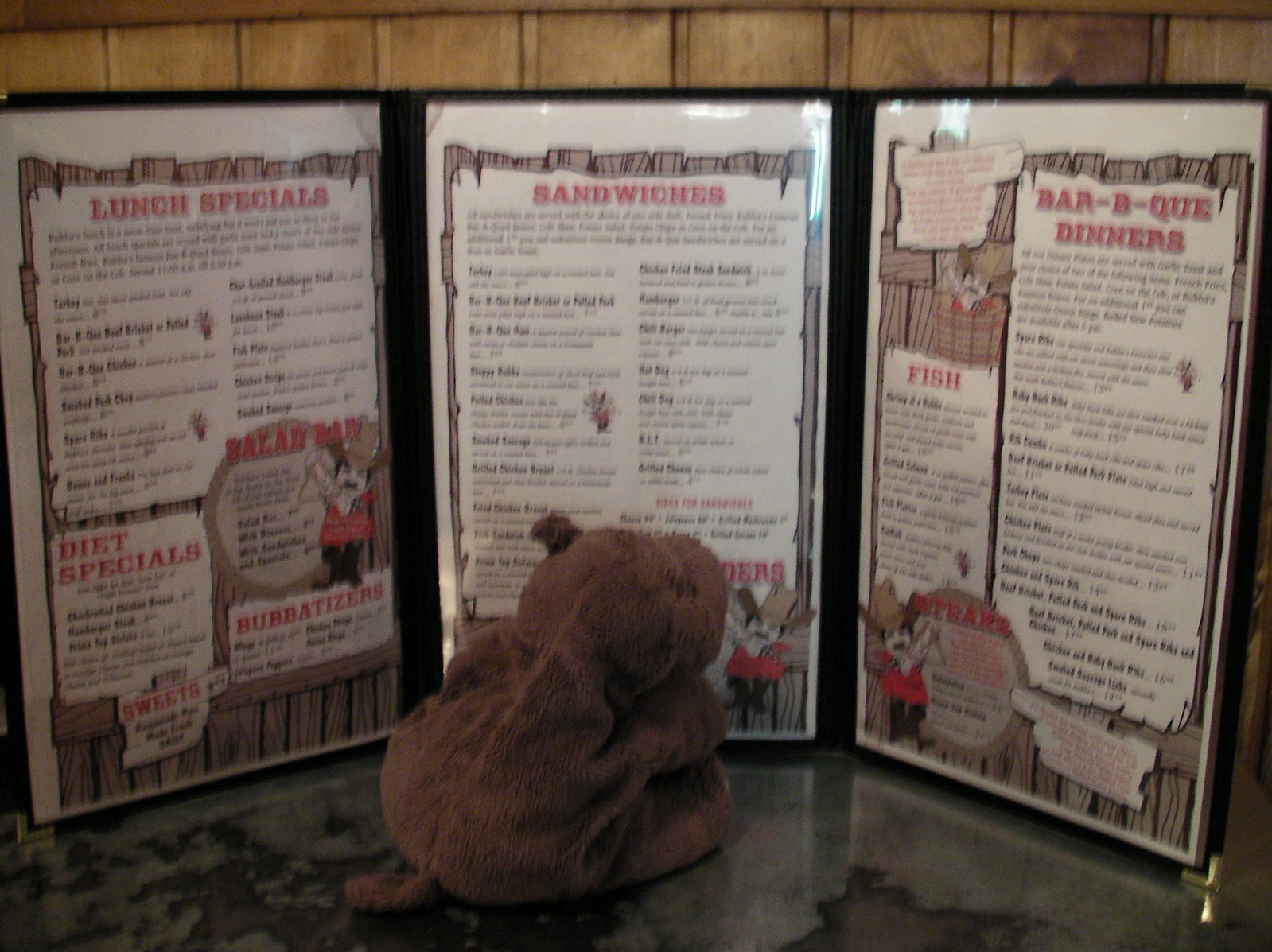The photograph captures a slightly blurry image of a three-paneled restaurant menu with a black-paneled body, resting on a gray countertop surface speckled with brown splotches. Positioned in front of the menu is a brownish stuffed animal. The background features a light wood-colored wall, adding a warm tone to the scene.

The menu itself is decorated with a brown fence graphic and showcases a cartoonish man character dressed in a red shirt, dark pants, and a light-colored hat, appearing throughout the panels. The first panel highlights "Lunch Specials" in red with a list of meal options in black font. It includes sections for a salad bar (in red), diet specials (in red) with corresponding options listed in black, "Bubba-tizers" (in red) with items listed underneath in black, and "Sweets" (in red) with dessert options listed below in black.

The middle panel is dedicated to "Sandwiches" (in red) and lists a variety of sandwich options in black, though the text is too blurry to read the specifics.

The final panel showcases "Barbecue Dinners" (in red) with various specials and their prices listed in black. This panel also features a section for "Fish" (in red), detailing a variety of fish-related specials in black.